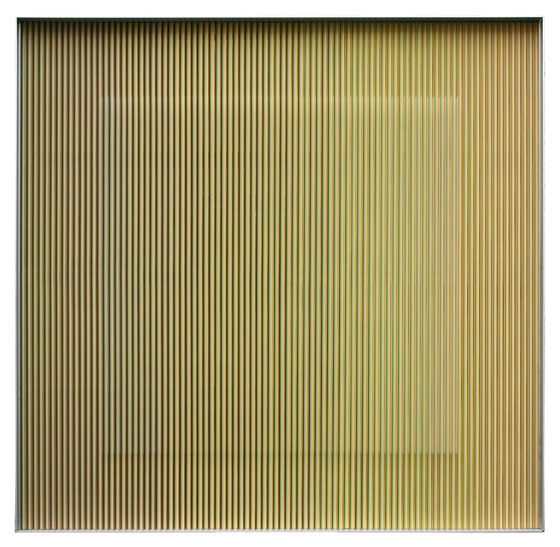The image displays a tan or beige-colored surface, resembling a window shade or vent, covered in extremely tight vertical lines spaced narrowly across the entire surface from top to bottom. The lines vary slightly in color, exhibiting hues of blue, purple, yellow, and white, with notable yellowish and white hues especially prominent on the right side. In the center of the image, if viewed from a distance, there appears to be a slightly raised square, differentiating itself subtly from the rest of the vertical lines. The top of the image features a horizontal strip of darker shading. The entire surface spans an estimated 12 to 15 feet in both width and length.